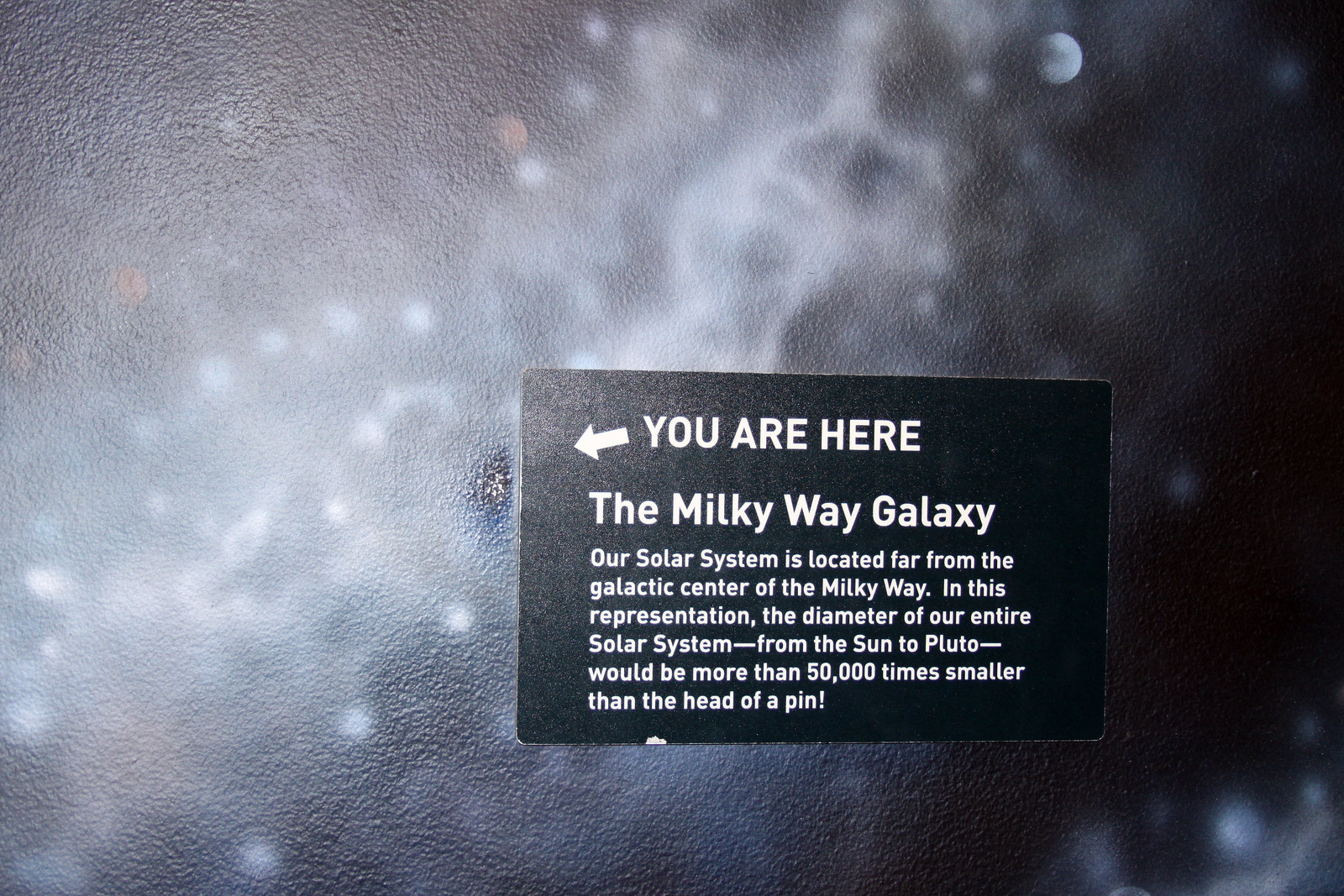The image is a detailed illustration of the Milky Way galaxy, primarily in black and white. The galaxy itself is rendered in white tones against the black background of space, interspersed with representations of gas clouds, dust clouds, and a few indistinct planets. Overlapping this galactic depiction is a black rectangular strip featuring white text. The text begins with an arrow pointing to a specific spot on the galaxy and reads, "You are here, the Milky Way galaxy. Our solar system is located far from the galactic center of the Milky Way. In this representation, the diameter of our entire solar system from the Sun to Pluto would be more than 50,000 times smaller than the head of a pin." The overall image appears to be from a planetarium or a similar educational display, though it is somewhat obscured by a glare from an external light source, making the detailed background slightly challenging to see. The rectangular strip with the text seems affixed onto the main illustration, providing a palpable context for the galaxy's vastness relative to our solar system.